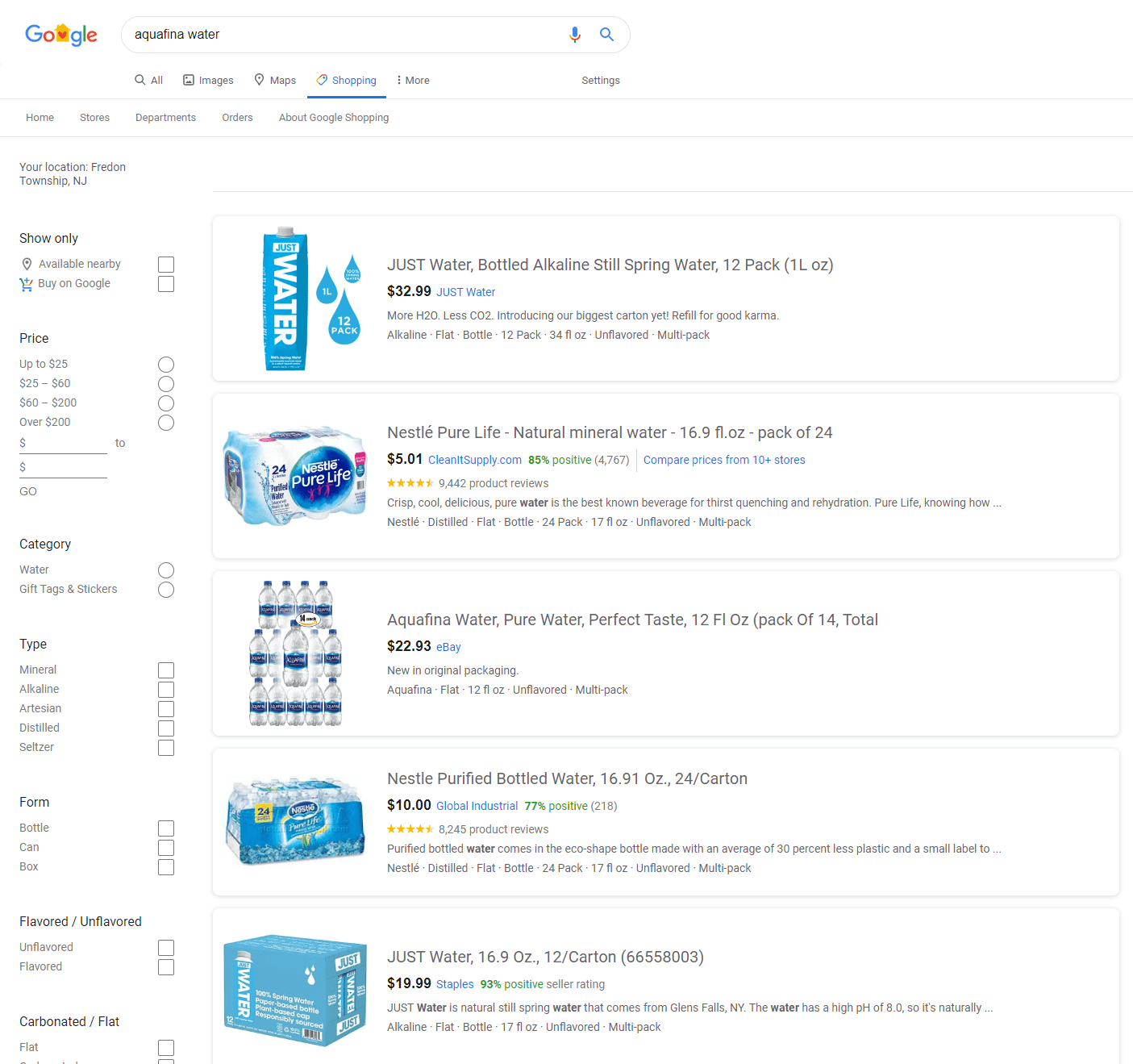In the image, a Google search page is displayed, focusing on the query "Aquafina water." The interface includes various tabs such as All, Images, Maps, Shopping (which is currently highlighted), More, and Settings. Below these tabs, different products are listed with their respective prices and details.

1. **Top Result**: 
   - **Water**: Priced at $32.

2. **Second Result**: 
   - **Nestlé Pure Life Natural Mineral Water** 
   - **Quantity**: 16.9 fluid ounces per bottle, sold in a pack of 24.
   - **Price**: $5.91.

3. **Third Result**: 
   - **Aquafina Pure Water, Perfect Taste** 
   - **Quantity**: 12 fluid ounces per bottle, sold in a pack of 14.
   - **Price**: $22.93.

4. **Fourth Result**: 
   - **Nestlé Purified Bottled Water**
   - **Quantity**: 16.9 fluid ounces per bottle, sold in a carton of 24.
   - **Price**: $10.

5. **Fifth Result**: 
   - **Just Water** 
   - **Quantity**: 16 ounces per carton, sold in a pack of 12.
   - **Price**: $20.

To the left of the product listings, there are various filtering options such as price, categories, types, forms, flavored or unflavored, and carbonated or non-carbonated waters. This reflects a search for Aquafina water, showcasing a comparison between different water brands and their prices in the Google Shopping tab. The background of the Google page is white, creating a clean and organized appearance.